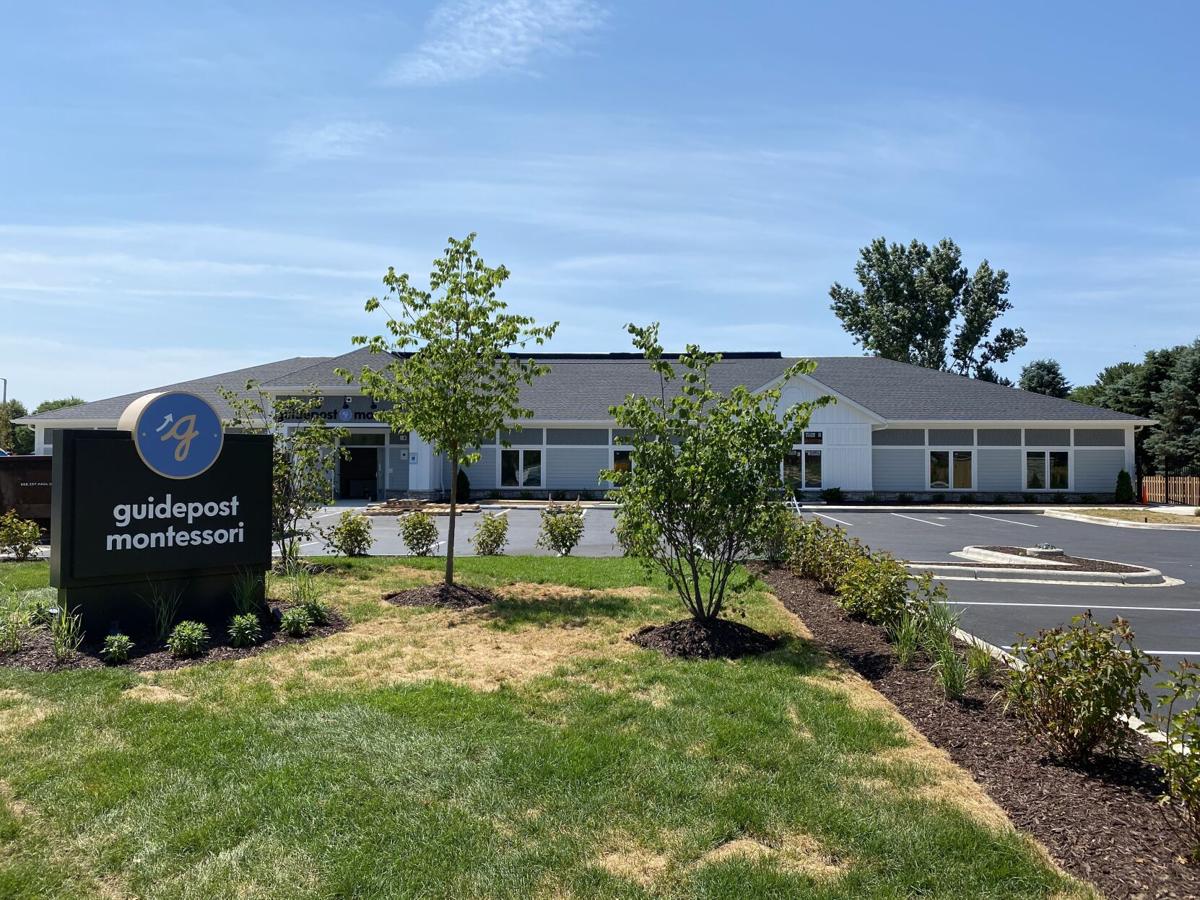The photograph showcases a light blue and gray single-story commercial building identified as Guidepost Montessori. The structure's roof is shingled in gray, and the front features a mix of white-trimmed windows and a large black or dark brown door. Notably, the tall, black sign in front reads "Guidepost Montessori" in white text, accompanied by a gold cursive 'G' within a blue circular background above, and is adorned with a white arrow curling around it. The sign is set amidst a variety of green plants and shrubs, some in mulch beds and others amidst patches of green and brown grass. On the left side of the building, there is a clear view of two double-paned windows framed in white wood and a partial view of another set, slightly obscured by two small green trees—one of which is more bush-like in shape. The front of the property features a large, empty parking lot with defined parking lines, beige separators with mulch and scattered plants. To the right of the building, a brown fence runs alongside with a row of dark green trees positioned behind it. The overall scene is set against a backdrop of a cyan sky accented with wispy white clouds.